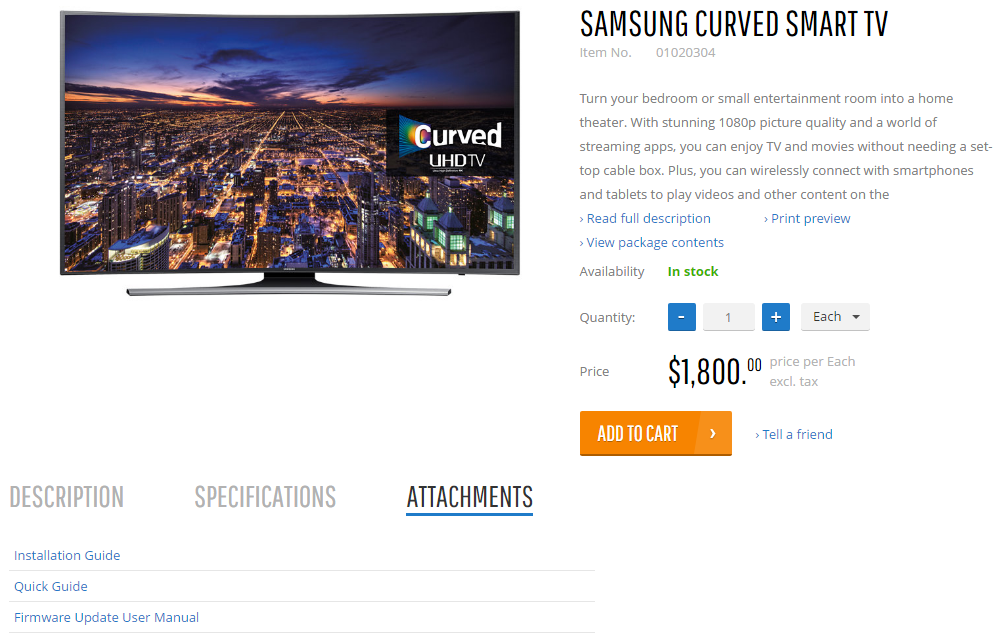The image is a screenshot of an advertisement for a Samsung Curved Smart TV. Prominently displayed in the upper left is a photograph of the TV, showcasing a beautifully lit cityscape at nighttime, with vibrant lights illuminating the scene captured from a distance. To the right of the TV image, a box highlights the text "Curved UHD TV." 

In the top right corner of the advertisement, the text reads "Samsung Curved Smart TV," followed by a marketing blurb: "Turn your bedroom or small entertainment room into a home theater with stunning 1080p picture quality in a world of streaming apps. You can enjoy TV and movies without needing a set-top cable box. Plus, you can wirelessly connect with smartphones and tablets to play videos and other content." 

The price for this high-definition home entertainment system is prominently listed as $1,800. An orange "Add to Cart" button is positioned for easy purchasing, accompanied by an option to "Tell a Friend."

Beneath the photo of the TV, there are three clickable options: Description, Specification, and Attachments, with Attachments currently selected. Under this section, several downloadable resources are listed: the Installation Guide, Quick Guide, and Firmware Update User Manual.